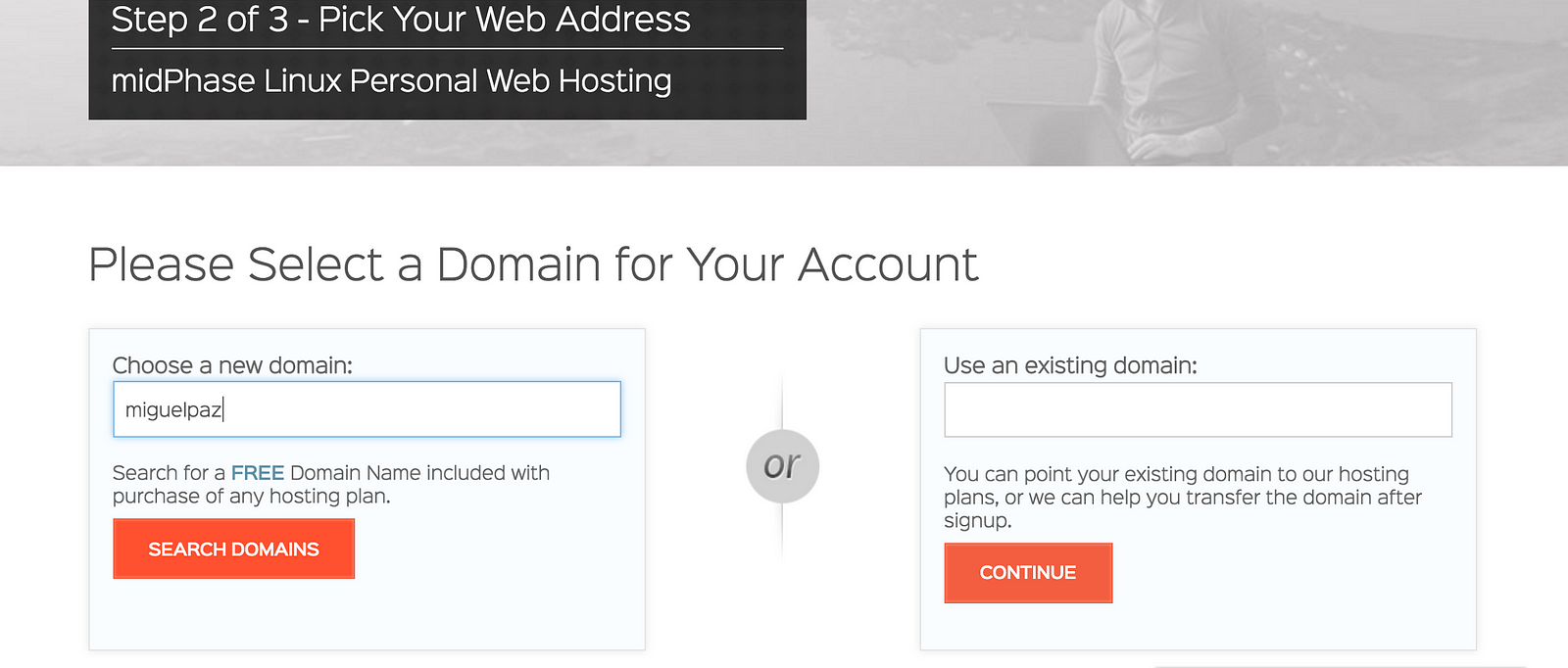The image is a wide rectangular banner, approximately twice as wide as it is tall. The top fourth of the image features a broad gray band stretching from left to right. On the right side of this gray band, there is a faint, light gray illustration depicting a person working on a laptop. Only their torso is visible, from the neck down to the waist, showing their left arm, hand, and chest, along with the back of the laptop.

On the left side of the gray band, within it, there is a dark black strip that contains two lines of white text. The first line reads, "Step Two of Three - Pick Your Web Address," with each word beginning with a capital letter. Below this line is a thin, horizontal white line. Underneath the line, in white capitalized letters except for the lowercase "mid-phase," it says, "Mid-Phase Linux Personal Web Hosting."

The remainder of the image has a white background. In large gray letters, it reads, "Please Select a Domain for Your Account." Below this, there are two distinct sections separated by a gray circle containing the word "OR" in capital letters.

The left section is enclosed by a light gray box. Inside the box, it says "Choose a New Domain," followed by a white input field outlined in blue. Below this input field, in blue capital letters, the word "FREE" stands out amidst the gray text, "Search for a free domain name included with purchase of any hosting plan." At the bottom of this section, there is an orange rectangle with white capital letters that read "SEARCH DOMAINS."

The right section, similarly outlined with a light gray box, is labeled "Use an Existing Domain." Below this, there is a wide white input field. Following the input field, gray text reads, "You can point your existing domain to our hosting plans, or we can help you transfer the domain after sign up." At the bottom of this section, there is an orange rectangle with white capital letters that say "CONTINUE."